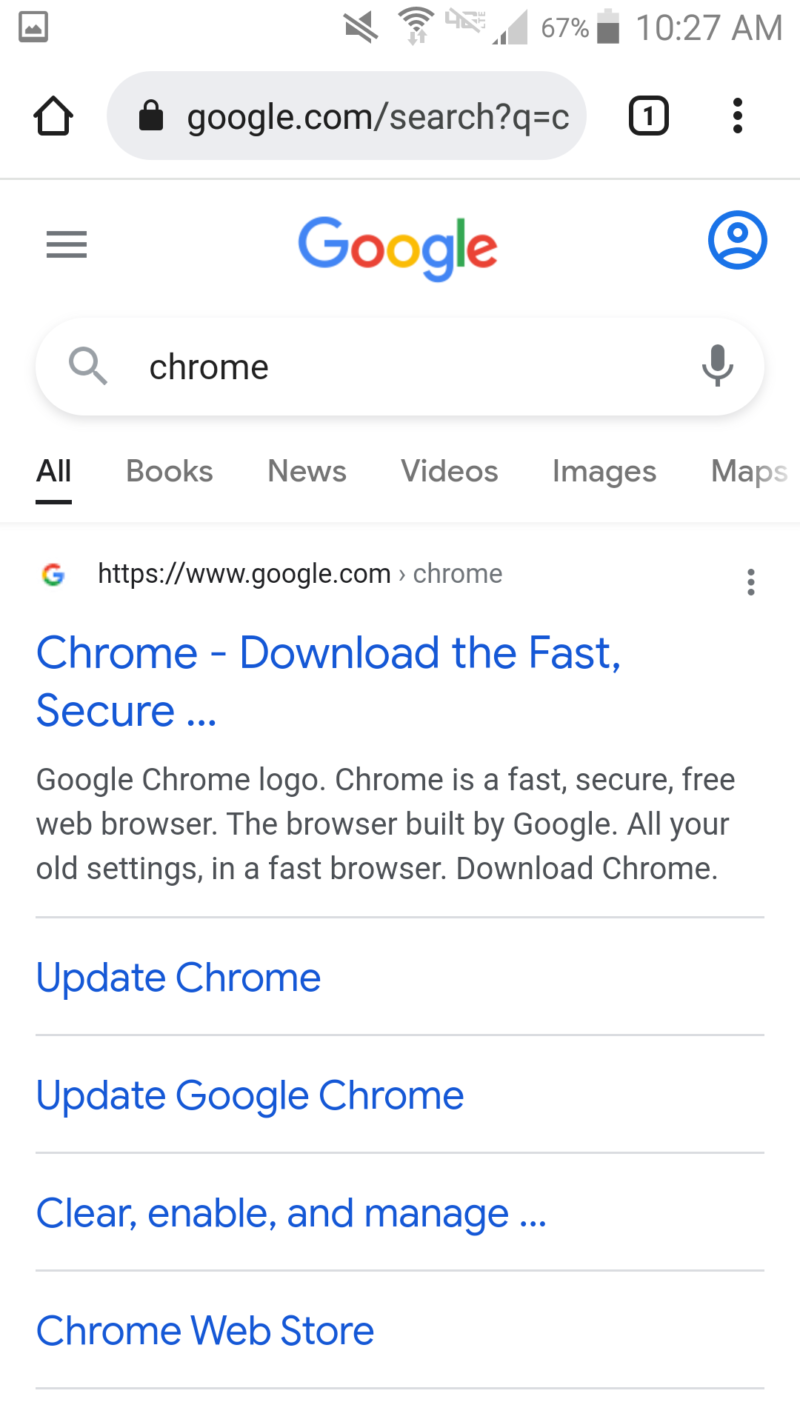The screen displays a Google Chrome browser window. The time reads 10:27 AM, and the battery level is at 67%. In the top address bar is the URL “google.com/search?q=c”. On the left side of the address bar is a house icon, and on the right are a square icon with the number '1' inside and three vertical dots. There is also a hamburger menu icon, followed by the Google logo and a blue profile picture icon.

Below the address bar is the search bar featuring a magnifying glass icon on the left and a microphone icon on the right. The search bar also displays a drop-down menu with categories such as "All," "Books," "News," "Videos," "Images," and "Maps," with "All" highlighted in blue.

A set of search results follows, starting with a description of Google Chrome. It reads: "Chrome is a fast, secure free web browser. The browser built by Google, all your old settings in a fast browser. Download Chrome. Update Chrome." The phrase "Download Chrome" and "Update Google Chrome" appears in blue text. Additional information includes "clear, enable, and manage," and references to the Chrome Web Store.